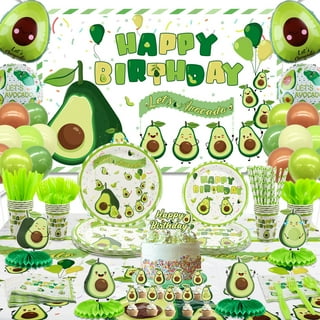The image showcases an avocado-themed birthday design centered around the phrase "Happy Birthday" written in various shades of green and yellow. The illustration is vibrant, featuring multiple cartoonish avocados with faces, some of which have humanoid characteristics. The avocados vary in size, with two prominently placed in the top left and right corners. Additionally, there's a festive array of party items including plates, cups, napkins, and streamers, all adorned with the same colorful “Happy Birthday” lettering and avocado motifs. The image also includes green-colored spoons, forks, knives, and straws. Towards the bottom center, a small birthday cake is featured, decorated with white icing, rainbow-colored sprinkles, and a top adorned with an avocado and the "Happy Birthday" message. Surrounding the cake are small avocado characters standing on a ribbon-like platform. The overall impression is a lively and cohesive avocado-themed celebration setup.